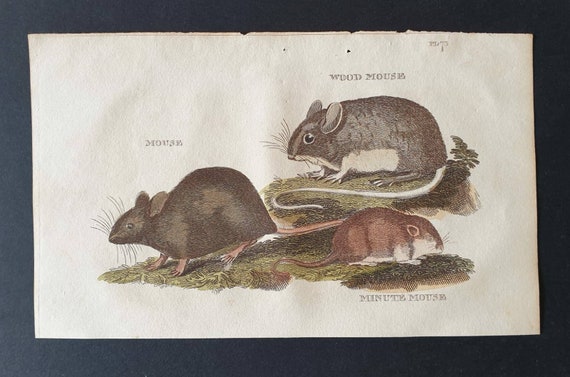This rectangular illustration features three distinct types of mice: the wood mouse, the mouse, and the minute mouse, all presented on an off-white sheet with a grey-to-black gradient border, transitioning from left to right. Each mouse is depicted in a green grassy setting with some foliage. 

The wood mouse is distinguished by its gray fur, white underbelly and tail, white feet, and a white ring around its eyes. It's one of the larger mice and faces to the left in the illustration. The regular mouse is plain brown with no distinct coloration except for its pink tail and feet, and it also faces left. The minute mouse, the smallest of the three, has a brown coat with a cream-colored underbelly, pink ears, a brown tail, and is depicted facing right. Together, they portray a detailed study of these different mouse species against the minimalist grassy landscape.